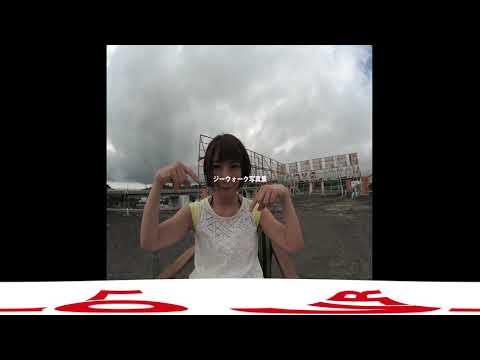This photograph captures a young Asian girl or possibly a teenager standing in an outdoor setting with a dreary, cloudy sky in the background, suggesting a somber mood. She has chin-length black hair with bluntly cut bangs and wears a cropped, short-sleeve or possibly sleeveless white and yellow shirt, with hints of a lime green undershirt underneath. Her arms are raised, with her hands pointing downward towards herself. The backdrop includes what appears to be a stadium and possibly additional buildings, with the entire scene framed by a black, computerized border measuring approximately 4x4 inches. Foreign letters, difficult to decipher, are imprinted or present on both a stick she is holding and a red and white ribbon positioned near her. The ground beneath her looks like a concrete area, potentially a parking lot, while she stands on what may be a small bridge, though the exact details are unclear.